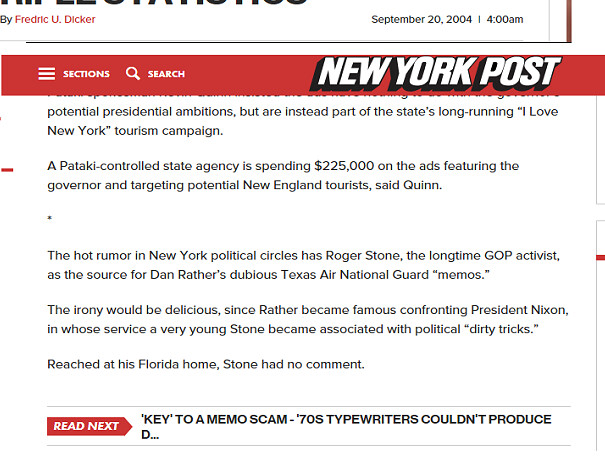The image is a screenshot of an article from the New York Post, dated September 20th, 2004, 4 a.m., and authored by Frederick U. Dicker. The website’s header includes a red banner with a menu icon and the word "Sections" on the top left, and a magnifying glass icon followed by the word "Search". On the right side of the banner, the bold white "New York Post" logo with a black drop shadow is prominently displayed.

The article mentions the "I Love New York" tourism campaign, overseen by a Pataki-controlled state agency, which is spending $225,000 on ads featuring the governor and targeting New England tourists. There is speculation within New York political circles about Roger Stone, a longtime GOP activist, being the source of Dan Rather’s disputed Texas Air National Guard memos. The article notes the irony stemming from Rather's rise to fame by confronting President Nixon, and Stone's early political connections with Nixon’s administration. When reached for comment at his home in Florida, Stone declined to respond.

Beneath the article, a section labeled "Read Next" teases the title of another article: "Key to memo scam: 70s typewriter couldn’t produce...".